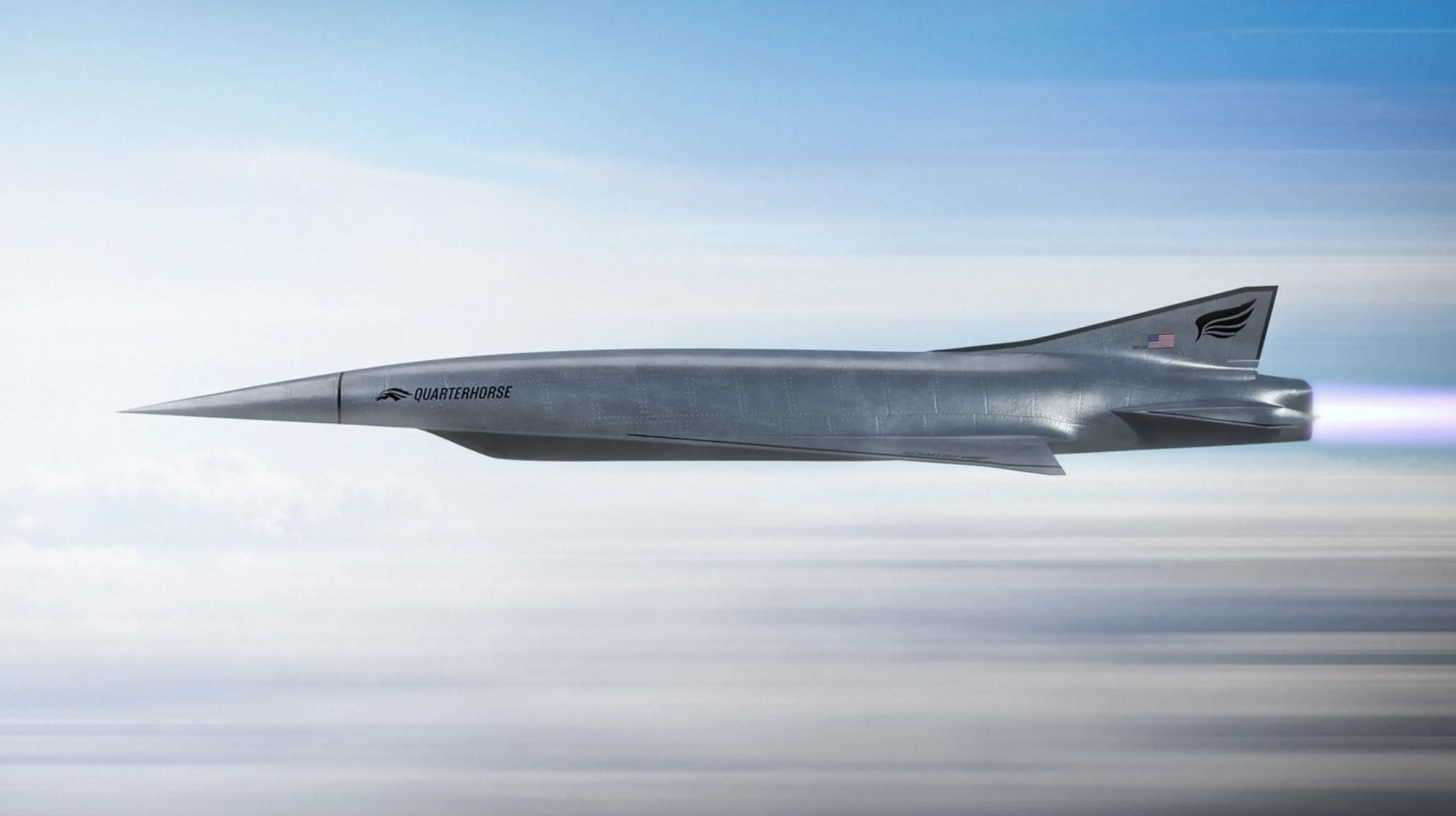This image, likely a conceptual rendering or partially edited photograph, features a sleek, modern jet resembling historic stealth planes but more advanced and streamlined. The jet has a long, cylindrical shape with no visible windows, marked by distinct metal rivets and seams on its stainless steel body. Its pointed nose transitions into an elongated fuselage with narrow, silver wings on its sides. The rear of the aircraft features two horizontal tail fins and a prominent vertical fin adorned with an American flag and a feather motif.

Emblazoned on the side of the jet is a logo depicting a horse's head accompanied by the label "Quarter Horse." This suggests the aircraft's identity. A striking feature of the image is the jet's exhaust, which is depicted as a vivid, purple-hued trail, enhancing the impression of high-speed motion. The background sky is blue with white streaks, resembling cloud trails that accentuate the jet's velocity. These visual elements collectively create a sense of immense speed and cutting-edge technology.